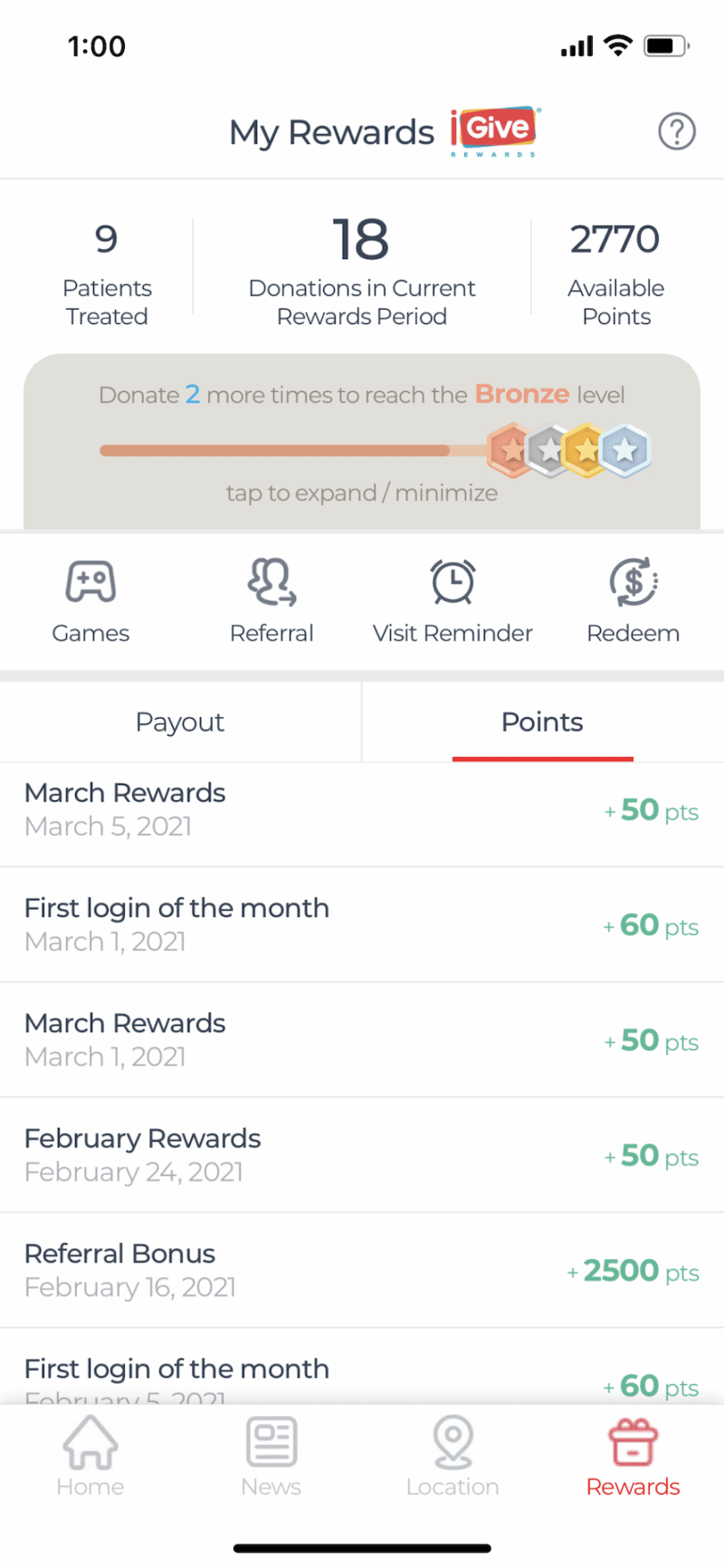The image display on the screen shows a comprehensive overview of a rewards program. At the top, the standard phone interface indicates the current time. In the center of the screen, the heading "My Rewards" is prominently displayed. Next to the heading, there is a red lowercase "i" icon, and a red background button with white text that reads "Give."

To the right, there is a question mark icon followed by detailed information about the user's rewards status:
- 9 patients treated
- 18 donations made in the current rewards period
- 2,770 points available

The message indicates that donating two more times will elevate the user to the bronze level. An interactive progress bar is displayed, showing the user's progression towards the bronze level. At the end of the progress bar, there are stars in various colors: red, grey, orange, and light blue, symbolizing different achievement levels.

Below this section, there are categories labeled "Games," "Referral," "Visit Reminder," and "Redeem." Further down, "My Rewards" is displayed again, followed by "First Login," and a historical log of the user's activities and progress within the rewards program.